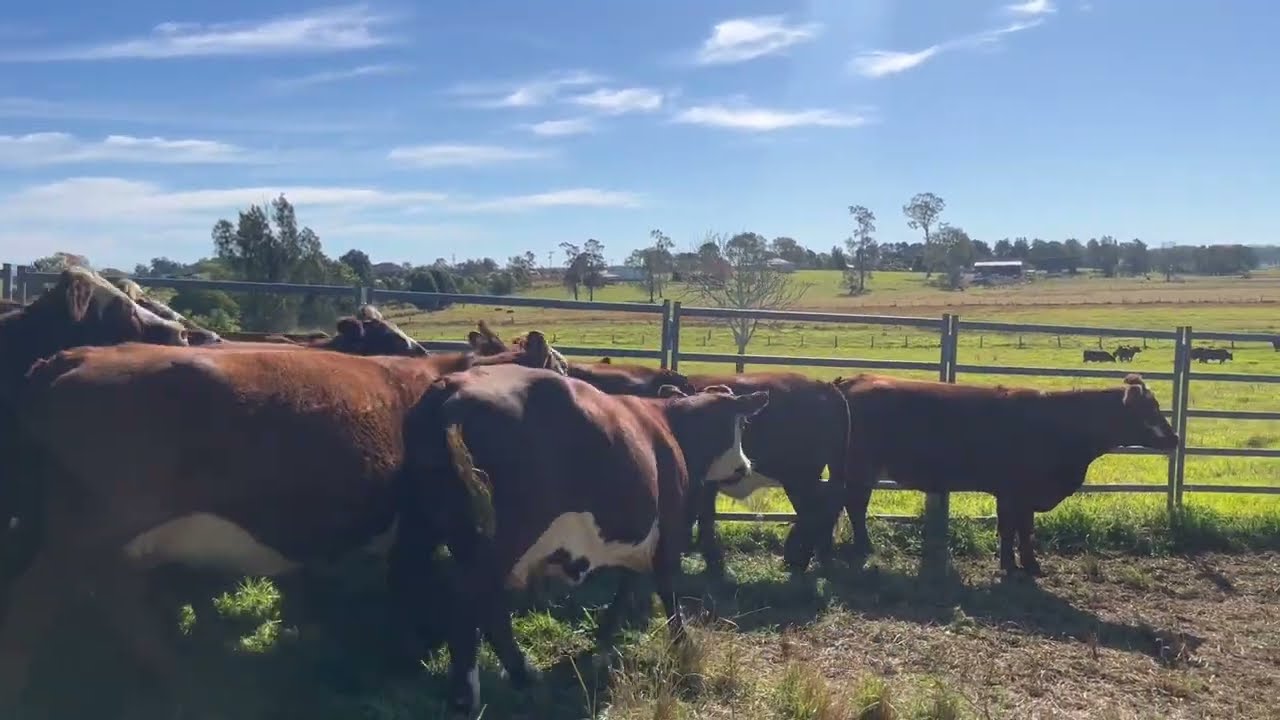The image captures a picturesque outdoor scene on a farm, with the main focus being around ten to fifteen brown and white cows in the foreground. These cows, some with distinctive white bellies, are standing in a partly eaten pasture, enclosed by a metal fence. They are all facing to the right, seemingly gazing longingly at the lush green pasture adjacent to them, which is separated by the fence. In the mid-ground, more cattle are visible within this greener pasture. A wooden fence runs behind this field, marking the boundary to a stretch of numerous trees. Beyond this tree line, there are several indistinct buildings which could be homes or farm structures. The sky above is a brilliant blue, adorned with sparse cirrus clouds, and the sun is shining brightly, casting shadows of the cattle in the foreground. The entire scene exudes a serene beauty of the countryside, highlighted by the peaceful disposition of the cows and the clear, sunny sky.